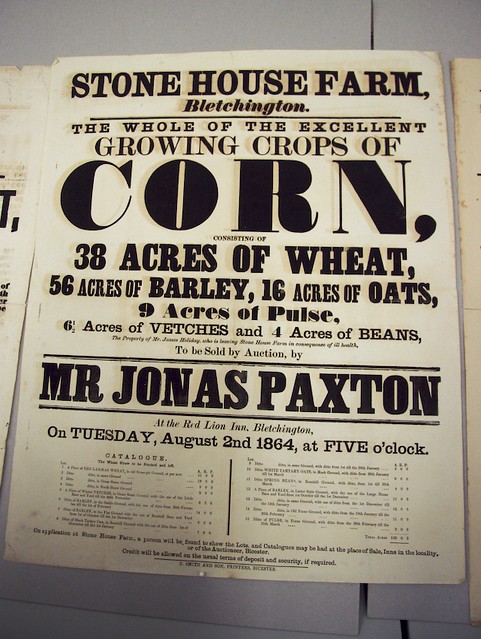The image features an aged, black and white handout resembling a vintage newspaper ad, displayed on a white-painted wooden surface. The handout's headline, in all capital letters, reads "STONEHOUSE FARM" with "Bletchington" printed below, separated by a thin black line. The main body of text, also in bold, declares "THE WHOLE OF THE EXCELLENT GROWING CROPS OF CORN," followed by a detailed list of the farm's produce: 38 acres of wheat, 56 acres of barley, 16 acres of oats, 9 acres of pulse, 6.5 acres of vetches, and 4 acres of beans. Additional, smaller text indicates that the crops are "To be sold by auction by Mr. Jonas Paxton at the Red Lion in Bletchington on Tuesday, August 2nd, 1864, at 5 o'clock." The handout includes more writing in small, unreadable print towards the bottom.